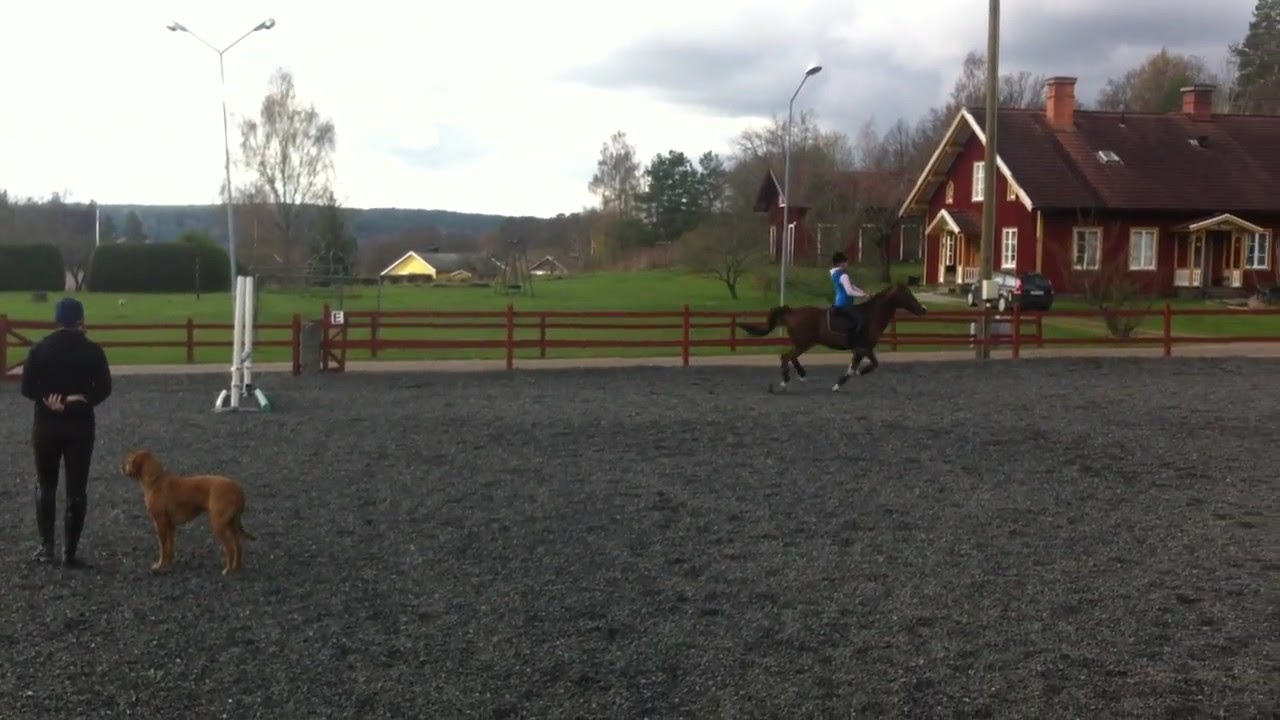This image, taken outdoors on an overcast day, depicts an equestrian scene within a menage. Dominating the upper right-hand corner, a red brick house, partially obscured by a treeline, hints at impending stormy weather with dark clouds gathering overhead. The left side of the sky remains slightly brighter, though still cloudy. 

The menage's ground is covered with fine gravel, an unusual choice for such an area, and is enclosed by a red or brown fence. To the left of the image, a man stands with his back to the camera, dressed in a long black shirt and pants, with his arms folded behind him. Adjacent to him, a large, reddish-brown dog mirrors his stance, also facing away from the camera. In front of this pair, a white jump post for horse jumping is visible.

On the right side of the frame, a dark brown horse with white socks, a black mane and tail, gallops away from the jump, ridden by a young person wearing a black helmet, white long-sleeved top with a hood, and a blue vest. The space behind is pastoral and dotted with greenery, featuring a black car parked in front of the red brick house, a dirt road, and additional distant rooftops peeking through the treetops. The overall ambiance of the photograph is filled with the charged quiet before a storm, capturing a moment rich with motion and anticipation.